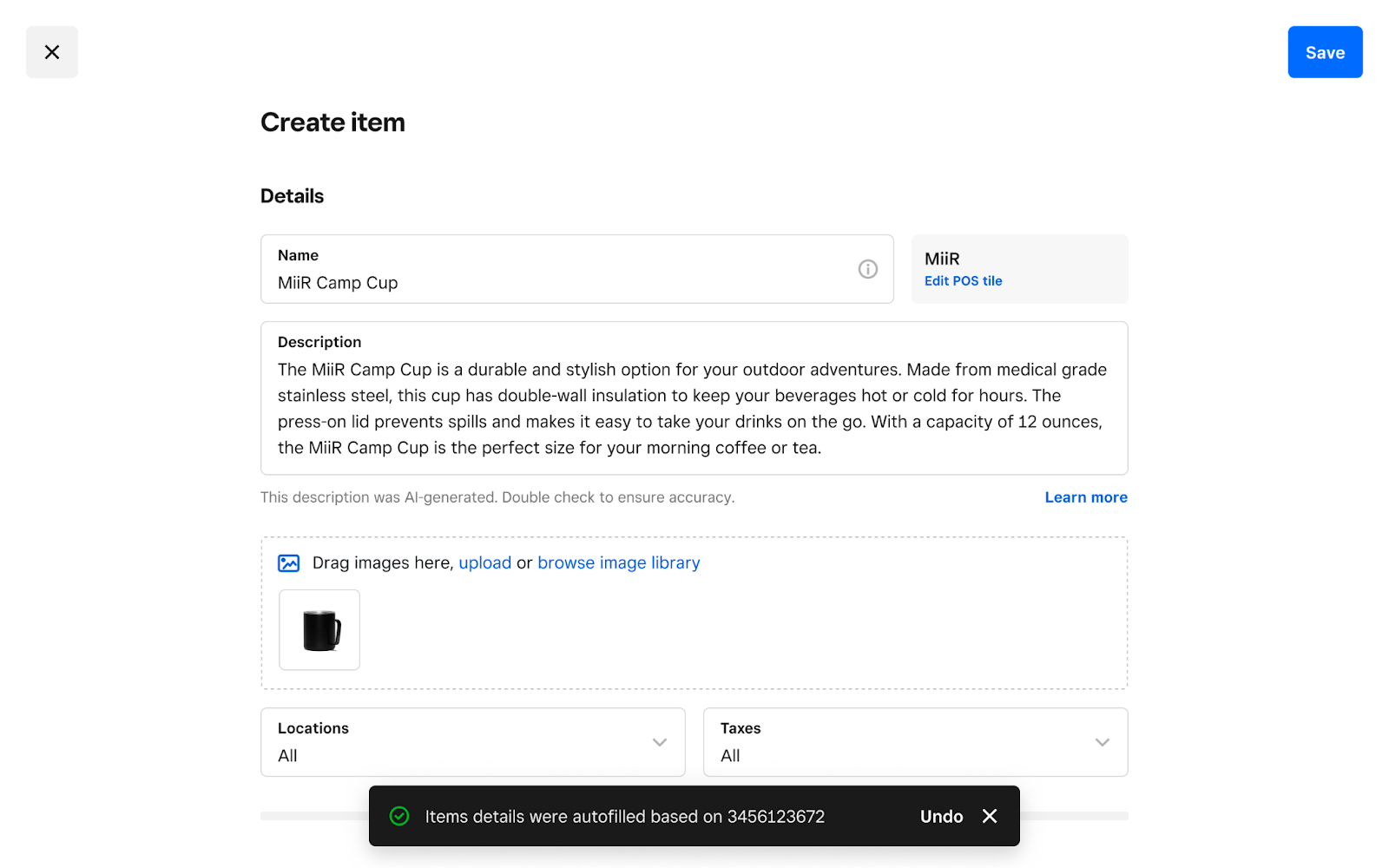This image displays a screen interface with a white background. In the top right corner, there is a blue "Save" button. Below that, two tabs are labeled "Create Item" and "Details." The first box contains a field labeled "Name," with the text "MIR Camp Cup" entered, accompanied by an information icon indicated as a small circle with an 'i' in it. Next, there is a light-blue box with the text "MIR edit pause title."

Following this, another box titled "Description" provides a detailed narrative about the "MIR Camp Cup." The description states that the cup is "a durable and stylish option for your outdoor adventures." It is made from medical-grade stainless steel and features double-wall insulation to maintain the temperature of beverages for hours. The description also highlights the press-on lid that helps prevent spills and makes it convenient for on-the-go use. With a capacity of 12 ounces, it is stated to be the perfect size for morning coffee or tea. Beneath this text, a disclaimer notes that the description is "AI generated, double check to ensure accuracy," with a "Learn more" link in blue text.

The interface also includes an image upload section with a light-blue box featuring a squiggly line and a dot, prompting users to "drag images here" or "upload or browse image library." This section has an image of a mug as an example. Below this, further input boxes are labeled "Locations" and "Taxes," each with drop-down menus labeled "All."

Towards the bottom, there's a black box with a green circle containing a check mark, which indicates, "Items details were auto-filled based on 3456123672." Adjacent to this, there are two buttons: "Undo" and an "X" button for closing or canceling actions.